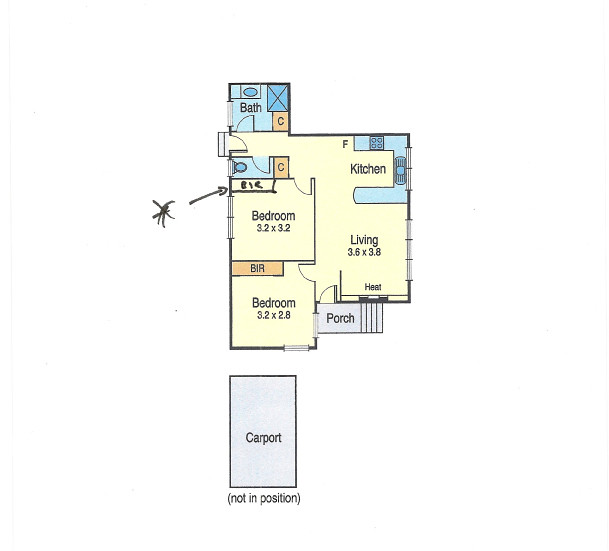This layout illustration depicts a detailed floor plan of an apartment, showcasing various rooms and amenities. At the top-left corner is the main bathroom, equipped with a shower and sink cabinet. Moving towards the right, the layout features a second bathroom, likely designated as the guest bathroom. Adjacent to this guest bathroom on the right-hand side, the kitchen is positioned, highlighted in blue. Below the kitchen, the living room area can be found, also marked in blue, and includes a heating unit. The living room extends to a porch area at the bottom center of the image.

On the left side of the layout, next to the guest bathroom, the first bedroom is situated, complete with an adjacent closet. Directly below this is the second bedroom. The bottom-right corner features a designated carport area for parking vehicles.

The floor plan is presented on a white background, with blue shading used to distinguish the bathroom, kitchen, and porch, while the remaining areas are left in white with black lettering for clear navigation and understanding.